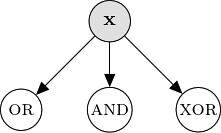This diagram, set against a white background, features a simple arrangement of circles, arrows, and labels. At the top center is a prominent black-outlined circle with a gray fill, marked with a bold black "X" in the center. Below, aligned along the bottom edge of the image, are three distinct circles in a row, each with a white center and black outline. 

The leftmost circle bears the label "OR" in black text. The center circle features the word "AND," also in black. The rightmost circle is labeled "XOR" in black lettering. 

Connecting these elements are black arrows: one extends from the 7 o’clock position of the top gray circle (with the "X") downwards to the "OR" circle. A second arrow directs from the center of the "X" circle straight down to the "AND" circle. Finally, from the 4 o’clock position of the "X" circle, an arrow points to the "XOR" circle on the bottom right. This structured flow clearly illustrates the relationships and connections between the labeled circles.